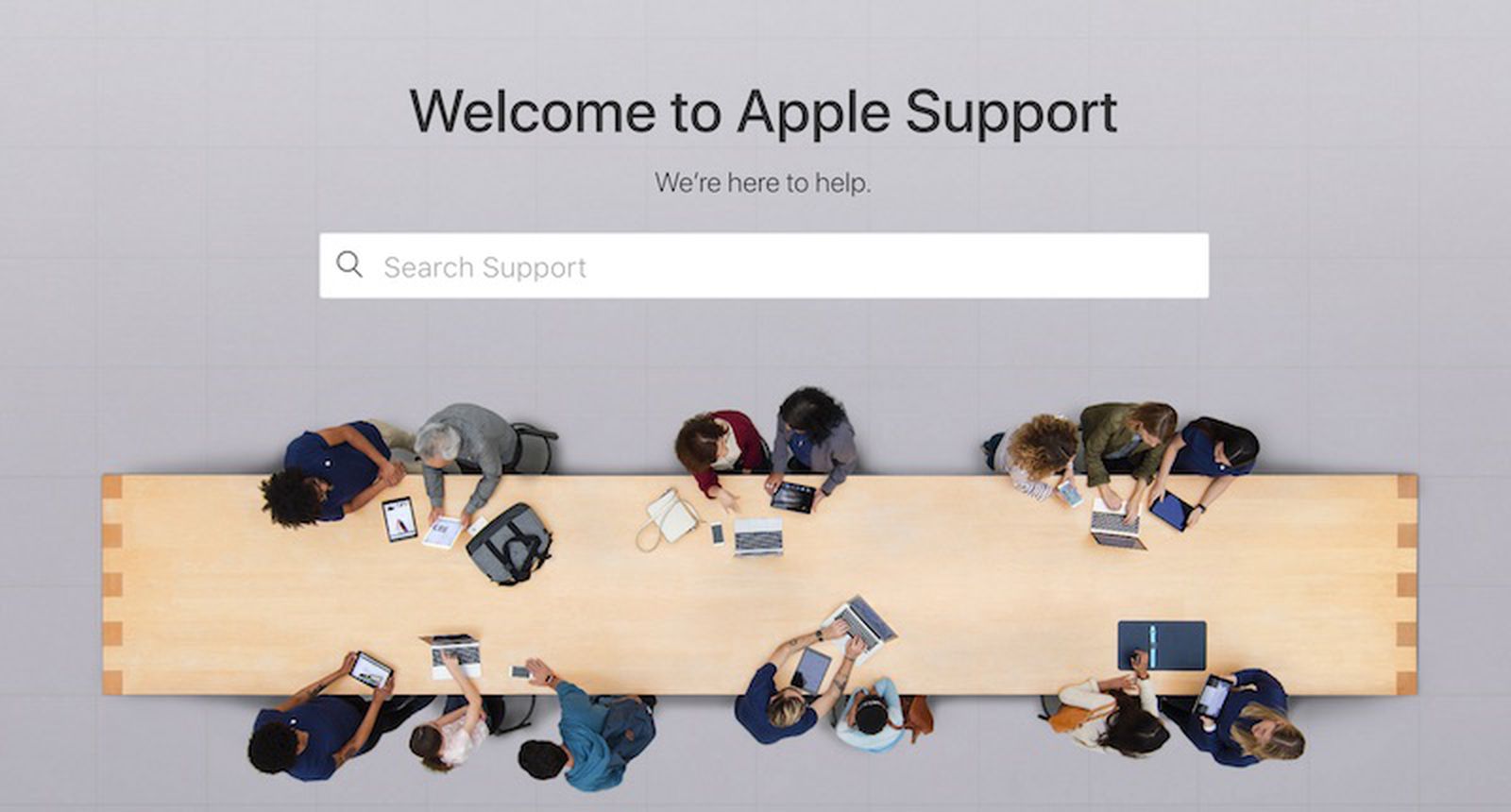The image depicts a vibrant scene from Apple's support webpage. The background is tastefully designed, featuring a warm, inviting theme. At the bottom of the image, there is a spacious table populated with multiple people engaged with various electronic devices, including computers and tablets. Specifically, there are three individuals grouped at the center-left of the table, flanked by two more people on the left side. Further along, on the right side of the image, there are three people closely huddled together, followed by two smaller groups of two. 

The table itself is a beige-brown color, accented by darker brown squares at each end, providing a modern and stylish touch. Above the scene, there is a large, white search box with the text "Search Support" inside, accompanied by a magnifying glass icon to the left. At the top of the image, welcoming text in black reads "Welcome to Apple Support," with the reassuring phrase "We're here to help" in slightly smaller, but equally bold, black letters just below it.

This image aims to convey the availability and approachability of Apple’s customer support, highlighting both the collaborative nature of assistance and the sophisticated design of the support portal.